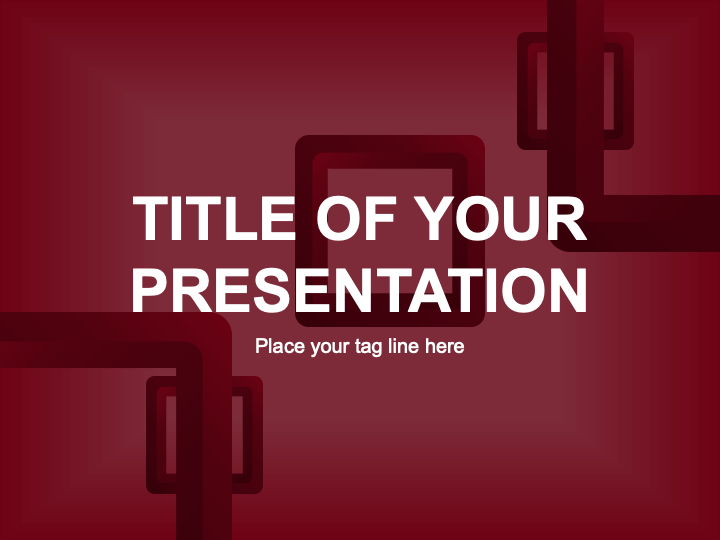This is a horizontal digital graphic design image primarily composed of maroon hues, with varying lighter and deeper shades of maroon creating a gradient effect that transitions from a lighter center to darker corners. In the very center of the image, bold, all-caps white text reads "TITLE OF YOUR PRESENTATION" while immediately beneath that, in smaller lowercase white text, it states "place your tagline here." The layout suggests that this design serves as a template for a presentation title slide. Behind the central text, a series of dark red shapes add depth and visual interest. These shapes form a pattern of three vertically aligned squares, extending from the lower left corner to the upper right corner. Additionally, large squares that look like they have been sliced to create L-shapes frame the bottom left and top right corners of the image, layering the visual elements to create a 3D effect. Overall, the design is minimalist, focusing on the interplay between the text and the geometric designs within the rich maroon backdrop.